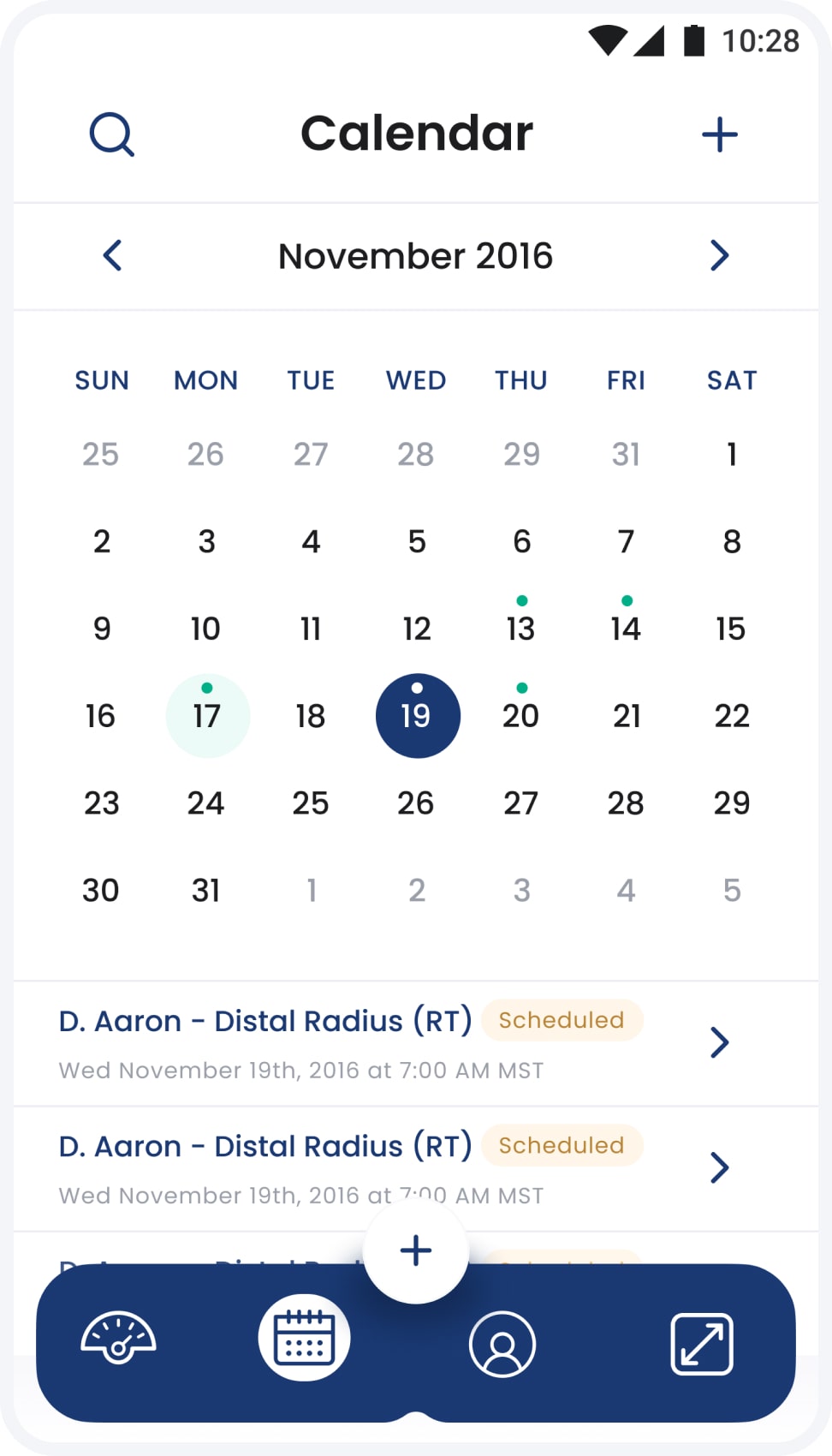Screenshot Description:

This is an image of a digital calendar interface. In the top right corner, the indicators show a full Wi-Fi signal, full data signal, and a full battery. The current time displayed is 10:28. 

Below the top bar, there is a search icon (magnifying glass) on the left, the word "Calendar" in the center, and a plus (+) icon on the far right. 

Further down, navigation arrows point to the left and right with "November 16th" displayed in the middle. 

The week row below starts with "Sunday" and ends with "Saturday." The dates are enumerated starting from 25 on a Sunday, proceeding to 31 on a Friday, and resetting to 1 on the following Saturday. The sequence continues from 2 to 8, then 9 to 15, and 16 to 22. A prominent blue circle highlights the date '19.'

Underneath the calendar, a text reads "D Aaron distal radius schedule" followed by another line simply stating "Schedule." 

The bottom bar features four icons: a speedometer, a calendar, a person, and a square with an arrow symbol indicating two hands. The bar itself is blue.